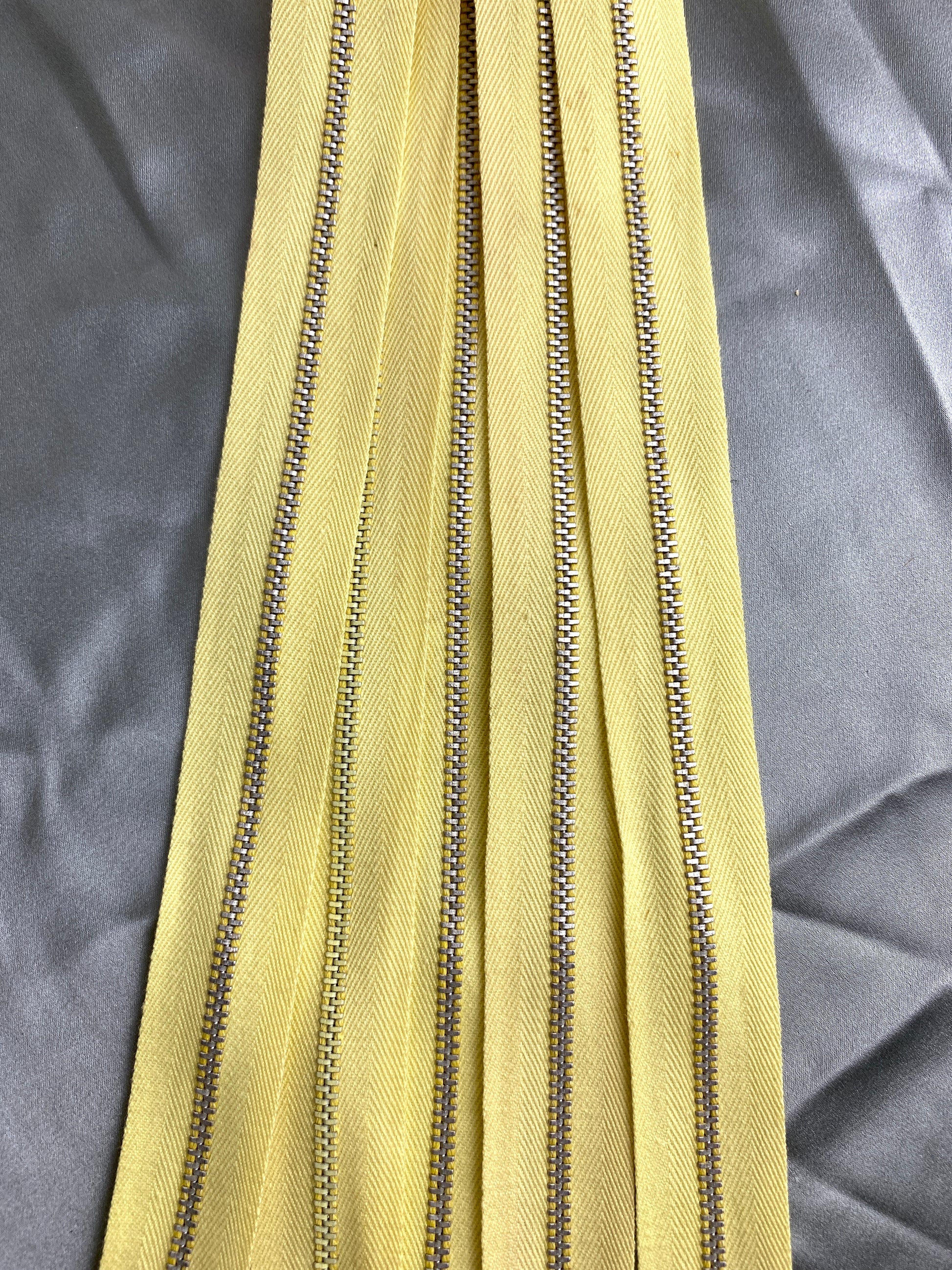This detailed photograph captures five zippers laid vertically and almost parallel, slightly overlapping each other as they fan out towards the bottom. Each zipper is aligned against a stripe of cream-colored fabric, resembling a yellow chevron pattern, with the zippers themselves displaying a shiny silver finish. The backdrop is a smooth, charcoal gray tablecloth exhibiting numerous imprinted folds and creases, notably one on the top left, two on the top right, and a jagged crease at the bottom right. The image, taken in a bright setting, is cropped tightly in a portrait layout, focusing on the central portion of the zippers and their accompanying cloth, and cuts off the top and bottom edges without fully revealing the ends of the zippers.